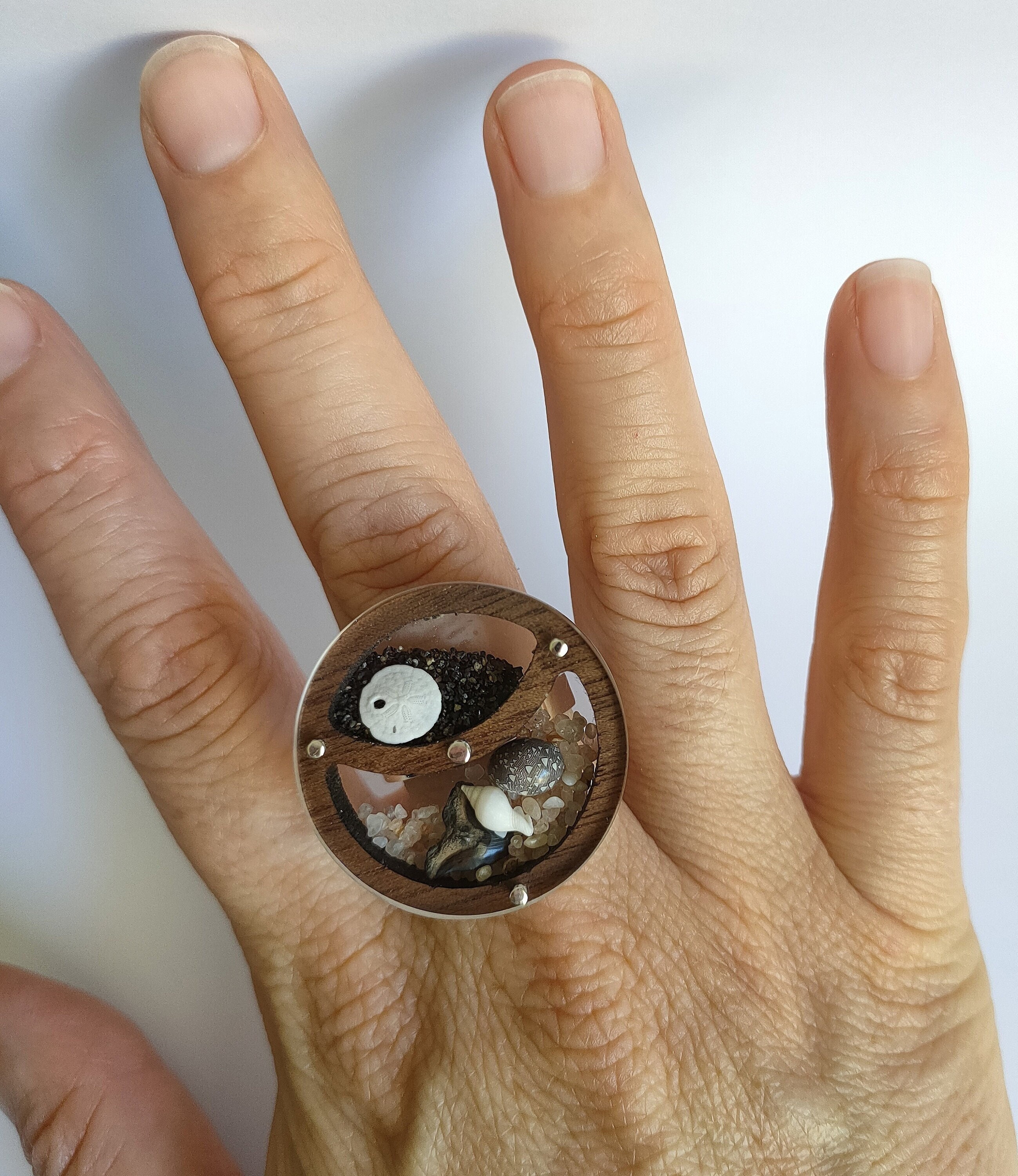The vertical, rectangular image captures a close-up of a white hand set against a light gray background with subtle shadows. The hand is angled from the bottom upwards to the left, with the fingers spread apart. Clearly visible on the middle finger is an intricate ring. The band of the ring is obscured, but its prominent design features a circular frame crafted from brown wood. Encased within this wooden frame is a transparent glass enclosure, revealing two distinct compartments. The upper compartment contains what appears to be black sand and a small, white sand dollar. The lower compartment, shaped like an upside-down arch or smile, houses tiny gray seashells, small white rocks, and additional shells in varying hues of gray, white, and brownish tan. Silver knobs affix the glass to the wood, providing additional detail to the craftsmanship. The fingernails in the image are a clear pink at the base, transitioning to a white tip, with visible veins and wrinkles on the knuckle area, adding a touch of realism to the scene.